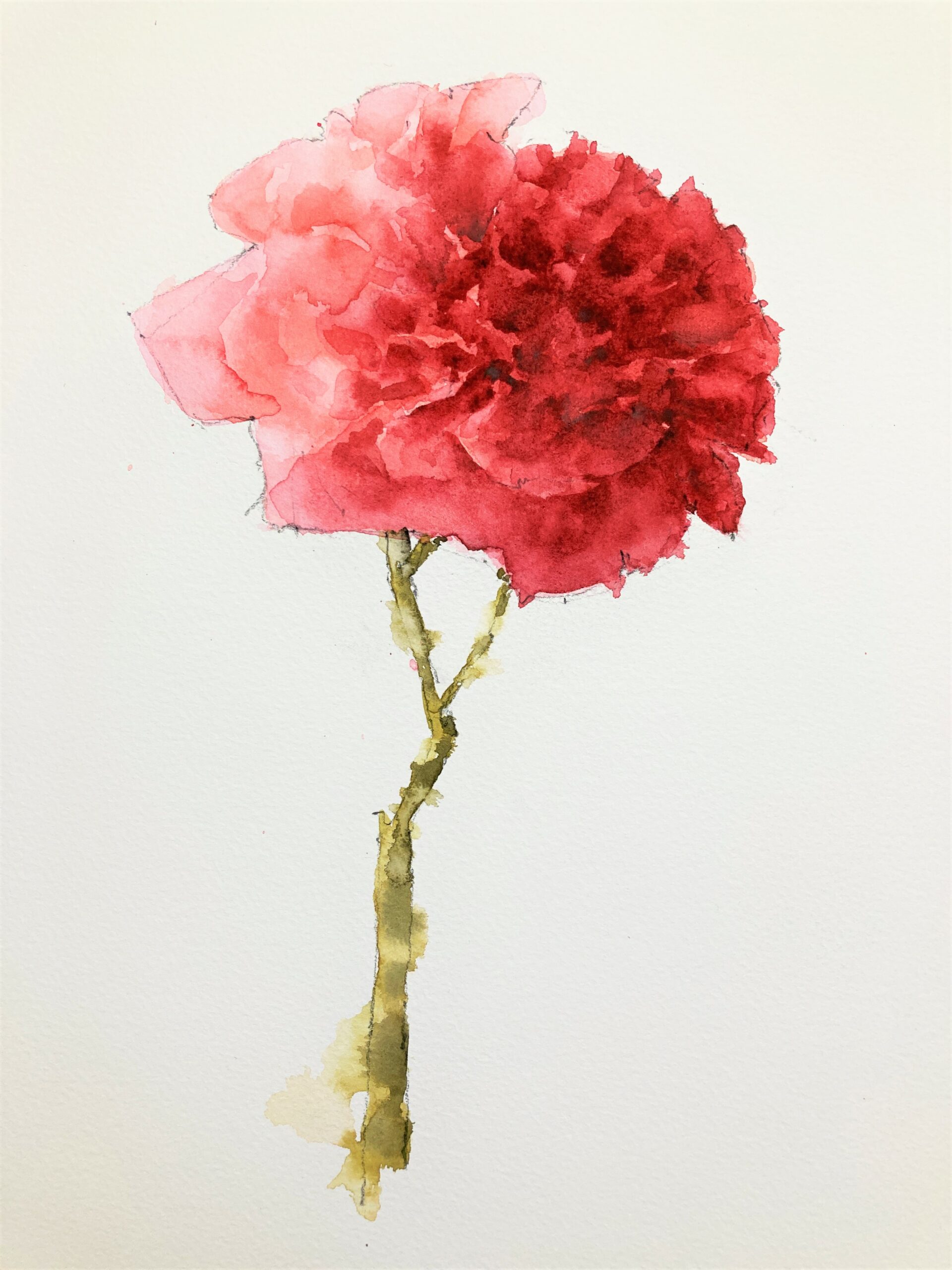This image showcases a detailed watercolor painting of a flower, reminiscent of a rose, featuring a vibrant blend of colors on an off-white, eggshell-like background. The flower's petals gradient from a darker red with touches of black on the right side to a lighter pink and white on the left, creating an effect as if meeting sunlight. The green stalk, outlined in black with hints of lighter green paint, extends from the bottom to support the elaborate bloom. The artist has achieved a realistic, almost tangible quality in the painting, with the watercolor seeping through lines and edges delicately, contributing to the lifelike portrayal of the rose-like flower.